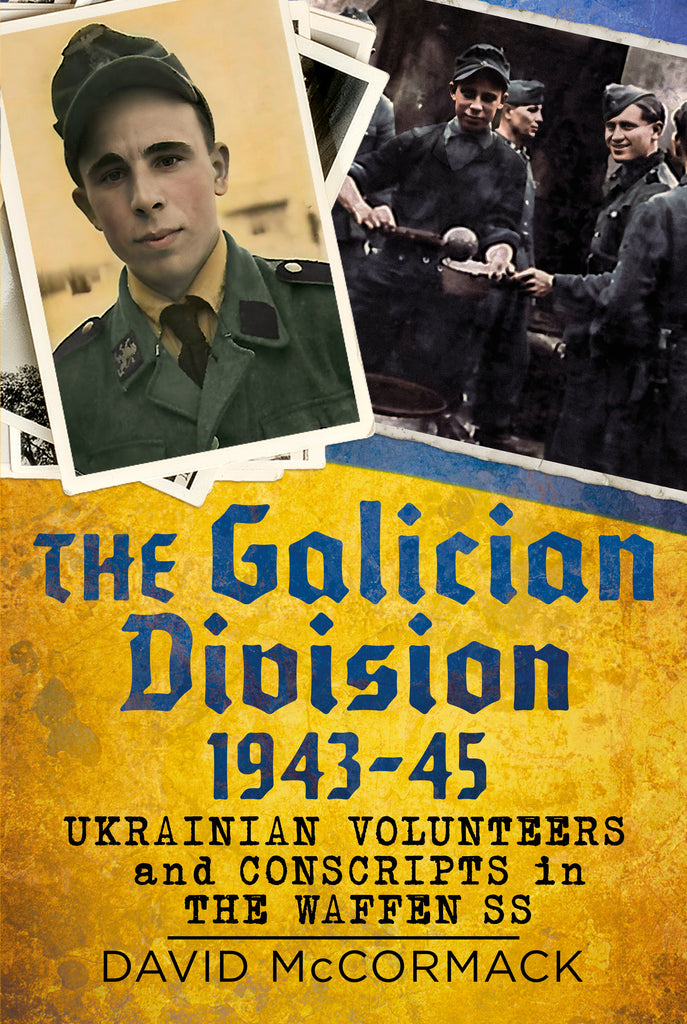This detailed poster, serving as a military advertisement, prominently features the title "The Galician Division 1943-1945" in large blue text, followed by smaller black text stating "Ukrainian Volunteers and Conscripts in the Waffen-SS" and the author's name, David McCormack, underneath. The poster's background primarily employs yellow and blue hues, reflecting the colors of the Ukrainian flag. 

At the top of the poster are overlapping printed photos, highlighted by a colorized portrait of a serious young boy in a green military uniform with black accents, a yellow shirt, a dark tie, and a green cap. His thick, dark eyebrows are notable. To the right, another photograph shows a group of young boys in similar uniforms, visible as they engage in serving gruel to each other. This image reveals details of four children, three facing the camera and one with the back of his head showing. The overall aesthetic of the poster combines elements of yellow and brownish hues, giving it an aged appearance that complements the historical theme.